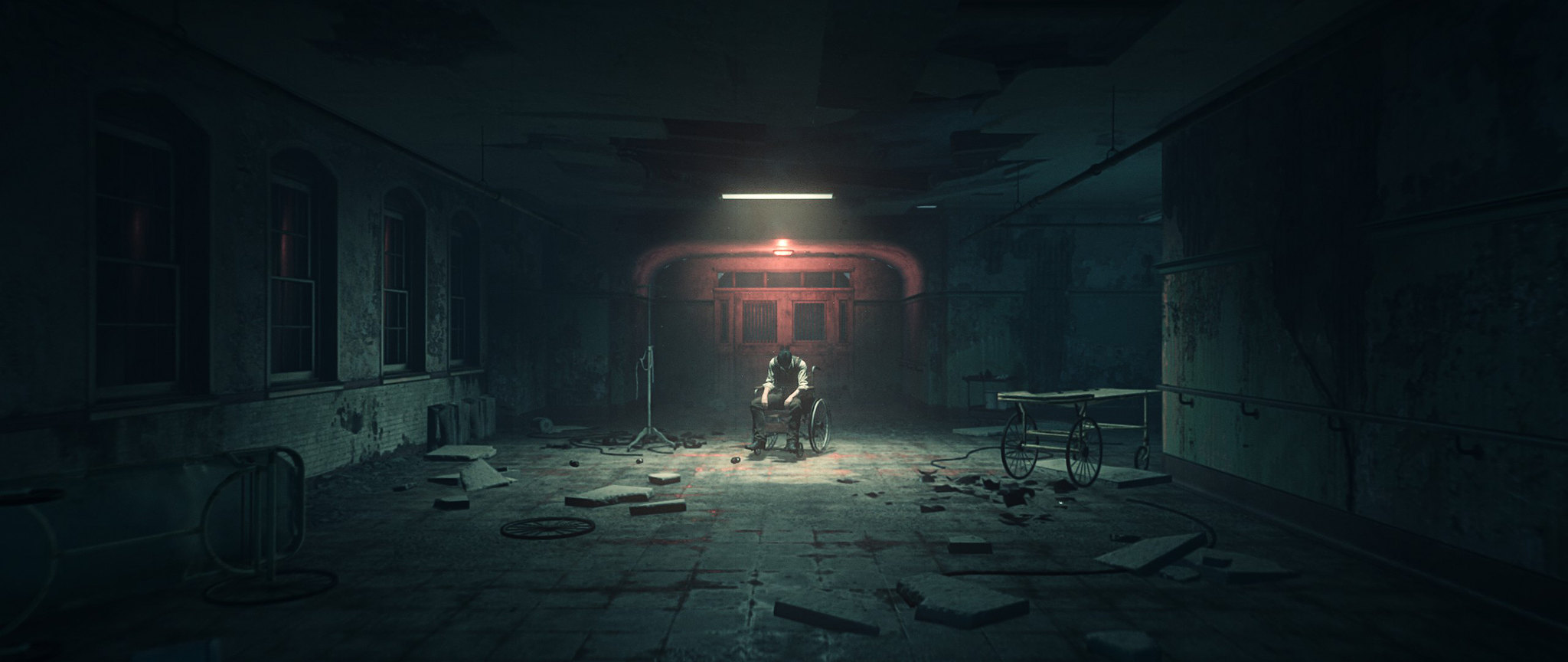The image appears to depict a grim scene, likely from a video game, set in a dark and dilapidated room that resembles an abandoned hospital, possibly a mental institution. The floor's tiles are disarrayed, and debris from the ceiling has fallen. The peeling paint and derelict environment add to the eerie atmosphere. Central to the scene is a figure in a wheelchair, partially obscured but identifiable by the visible arms and round wheels. To the left of the figure is an intravenous pole, and further to the right is an antique gurney with mismatched wheels. Above the figure, a fluorescent light faintly illuminates the scene. In the background, a grayish-red door with two windows stands out, marked by a glowing red emergency exit sign. Tall windows with a half-moon shape top adorn the left side of the room, adding to the dilapidated yet imposing ambiance.